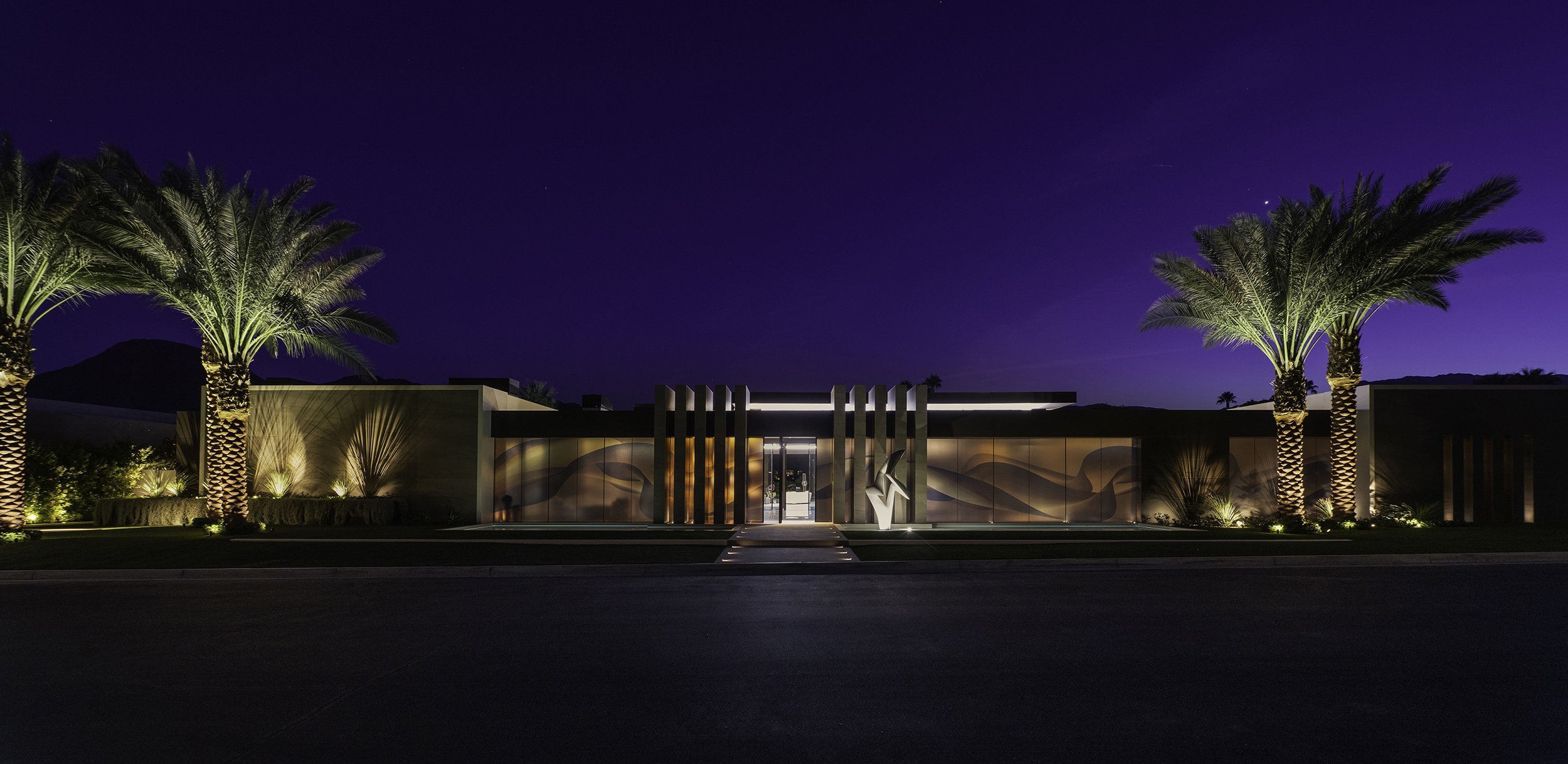The image captures a nighttime scene of a resort-like, single-story modern building with a flat roof, surrounded by a carefully illuminated landscape. The sky fades from a deep, dark blue to black at the top and transitions to a lighter purple towards the right side. There are five tall palm trees, two on the left and three on the right, framing the building and extending their lit branches over the roof, suggesting they are at least two stories high. The building's exterior features a lighted entry walkway and spotlights that accentuate the trees and the structure, creating dramatic shadows. Central to the façade is a door flanked by an abstract decorative fountain and statue. The photograph appears to be taken from across the street, adding a sense of depth to the nighttime ambiance.